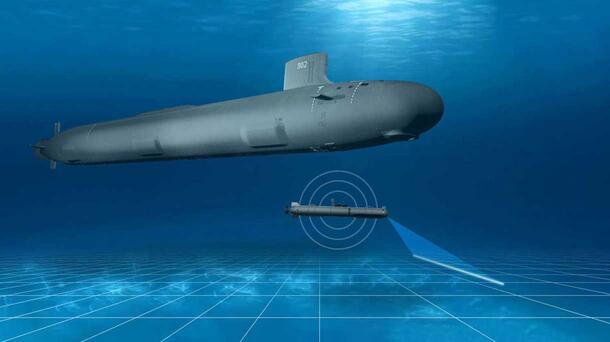This image is a detailed computer-generated rendering depicting an underwater scene. At the focal point is a long, pill-shaped gray submarine, oriented with its front end to the right and its back end to the left, situated just above the middle of the picture. The submarine features a fin on top, adding to its sleek, elongated bullet-like appearance. Below it, there is a smaller version of the submarine, possibly representing a missile, displayed within concentric spiraled circles, forming a radar-like pattern with a cone projecting ahead.

The majority of the image is composed of various shades of blue, signifying the underwater environment. The top section of the picture showcases the ocean's surface, where sunlight penetrates the water, creating ripples and a lighter blue hue amidst a predominantly darker blue background. In the center, the water gradates to a medium blue, while the bottom is characterized by a complex grid of light blue lines forming squares and rectangles against the darker blue ocean floor, further suggesting a video game-like environment. The combination of these elements creates a vivid and immersive underwater scene.